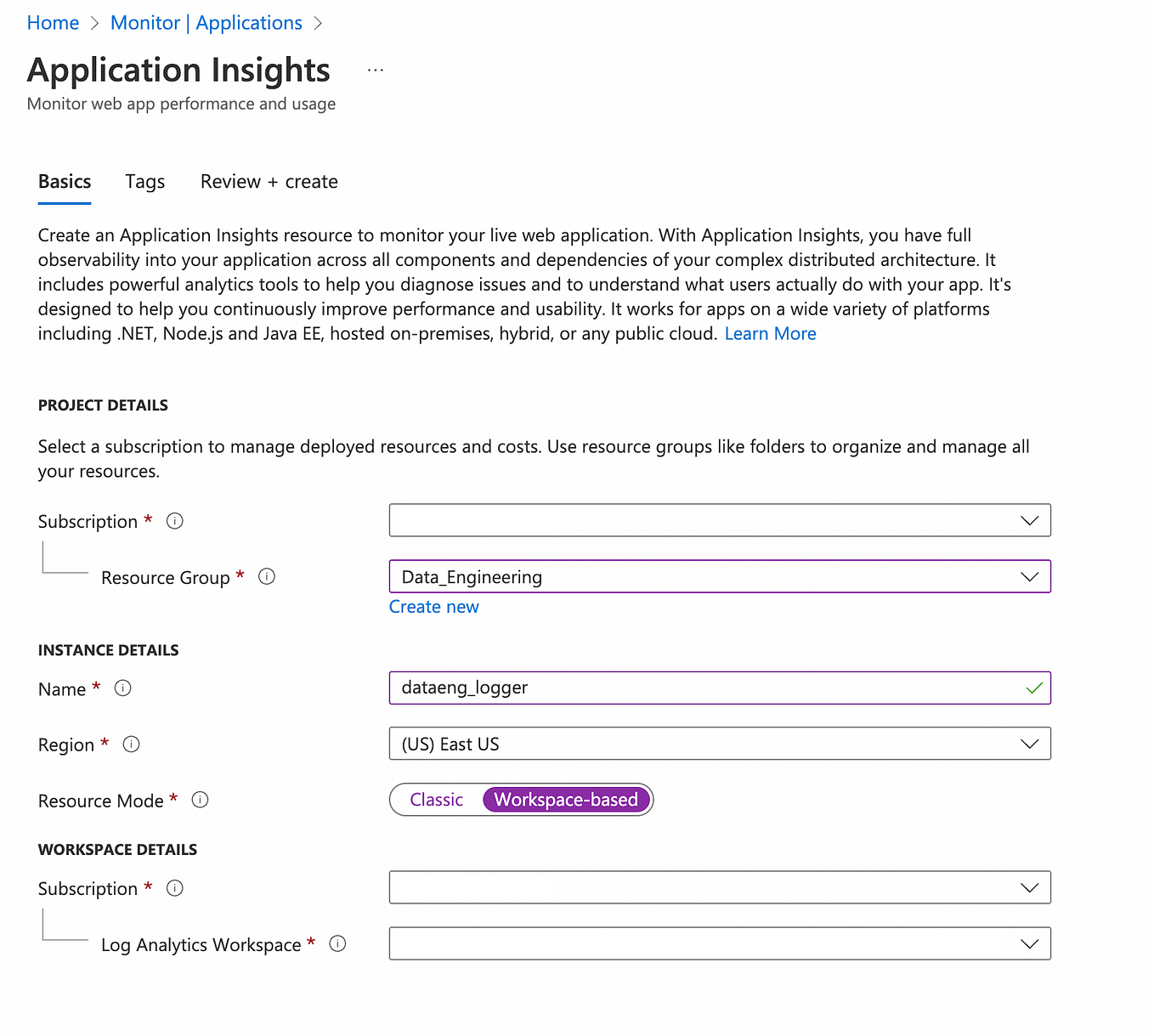This image is a detailed screenshot of an applications page with a clean, white background and black text adorned with blue hyperlinks. At the top left, "Application Insights" is prominently displayed. Above it, there are blue links for "Home," "Monitor," and "Applications."

On the left side, the page features a navigation menu with categories such as "Basics," "Tags," and "Review and Create." The "Basics" tab is currently selected, revealing informative text accompanied by a blue "Learn More" link. Below this section are "Project Details," which include areas for "Subscription Information" and "Resource Group."

Further down, "Instance Details" are provided, with fields for the name and region. There is also a resource mode slider, which offers two modes: "Classic" and "Workspace-based," with the latter highlighted in a purple bubble. 

At the bottom left, the "Workspace Details" section includes boxes for "Subscription" and "Log Analytics Workspace," each with a small gray down arrow for selection. Notably, the "Instance Details" name box features a green checkmark, indicating successful entry, while small red asterisks next to items in the left-hand column signify required fields.